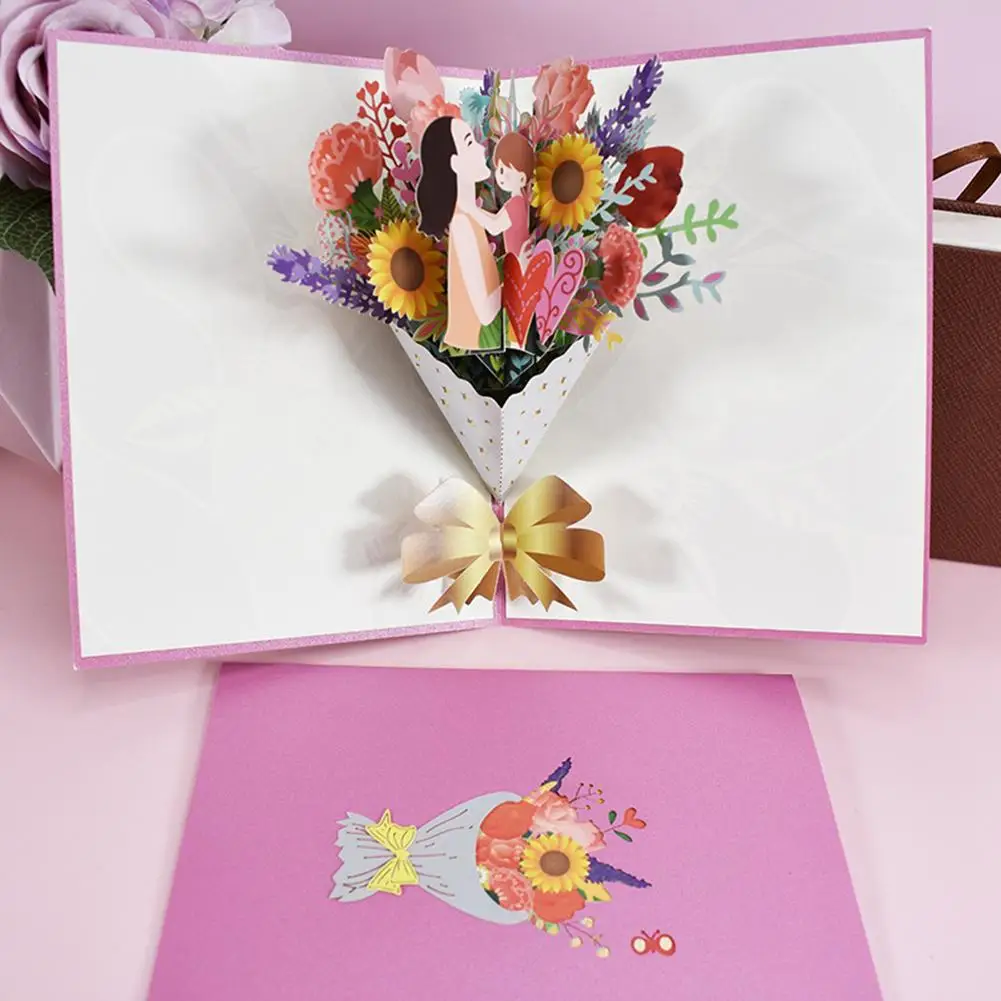This photograph features a detailed view of a pink greeting card designed with a 3D pop-up component. In the foreground, we see the card closed, showcasing a vibrant cover that highlights a bouquet of flowers, including sunflowers, roses, tulips, and other colorful blooms in shades of yellow, red, pink, and purple. Tied with a yellow bow, the bouquet is the main focus on the cover.

In the middle of the photograph, the card is opened to reveal a pop-up feature. This 3D element depicts a heartwarming scene of a mother with dark brown hair wearing a sleeveless shirt, holding her child who has light brown hair and a short-sleeved pink shirt. They are surrounded by the same types of flowers from the cover, arranged as if they are blooming from a white plant pot adorned with another yellow bow. This intricate artwork gives the impression of a shared, tender moment amidst a floral display.

In the background of the scene, we notice a light pink wall and some additional flowers, adding to the overall warm and welcoming ambiance. The open card stands upright, while the closed card lies in front, allowing viewers to appreciate both the inside pop-up artistry and the elegant cover design.